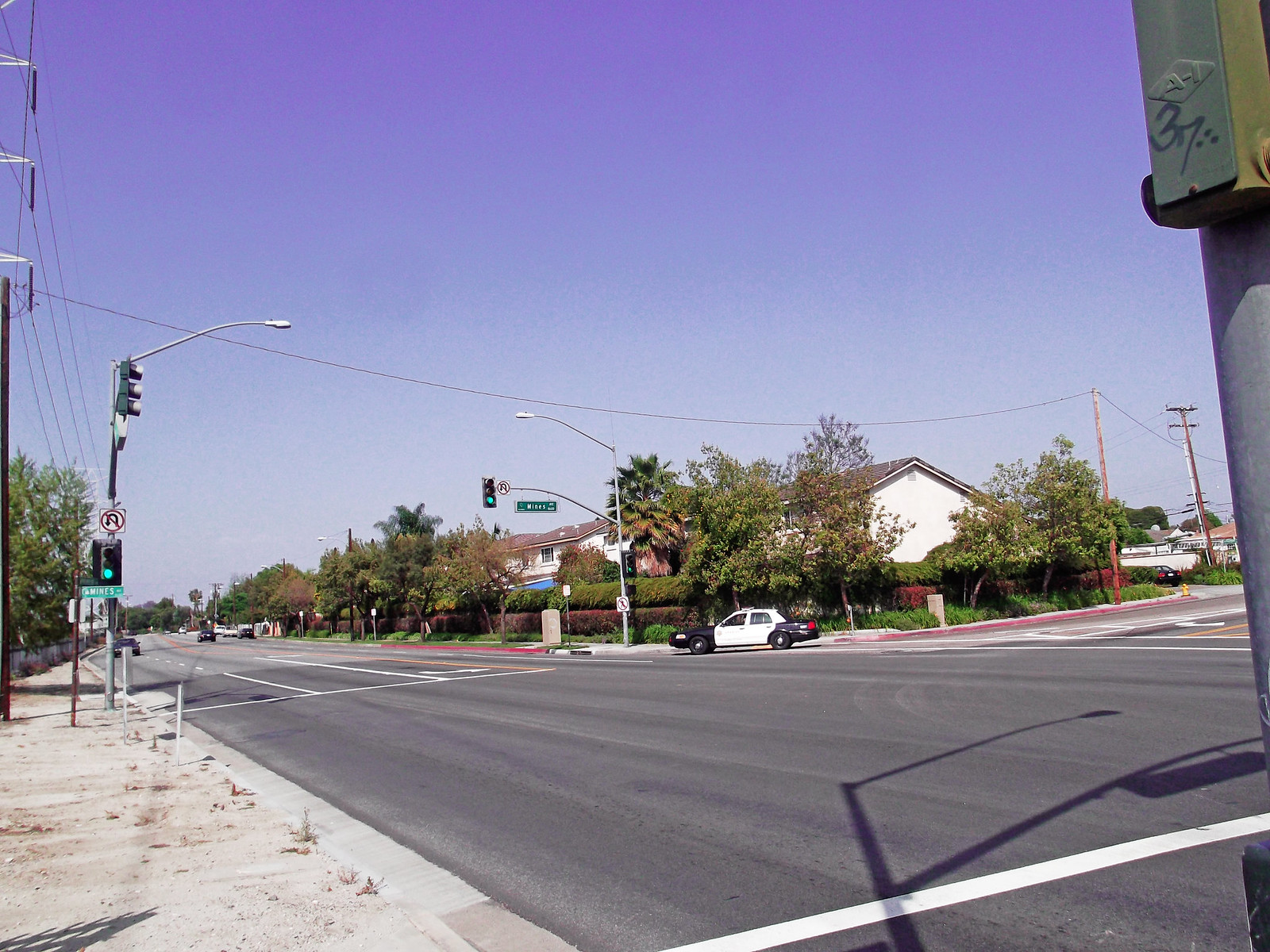This photograph captures a tranquil neighborhood intersection under a radiant, cloudless blue sky. At the center of the scene, a vintage police car, seemingly from the 1980s, is making a right turn against a green stoplight. The intersection is mostly deserted, with a few distant cars in the background. On the corner behind the police car stands a charming yellow house, partially concealed by a line of lush shrubs that serve as a natural fence. The scene evokes a sense of nostalgic calm, highlighting the timeless simplicity of suburban life.